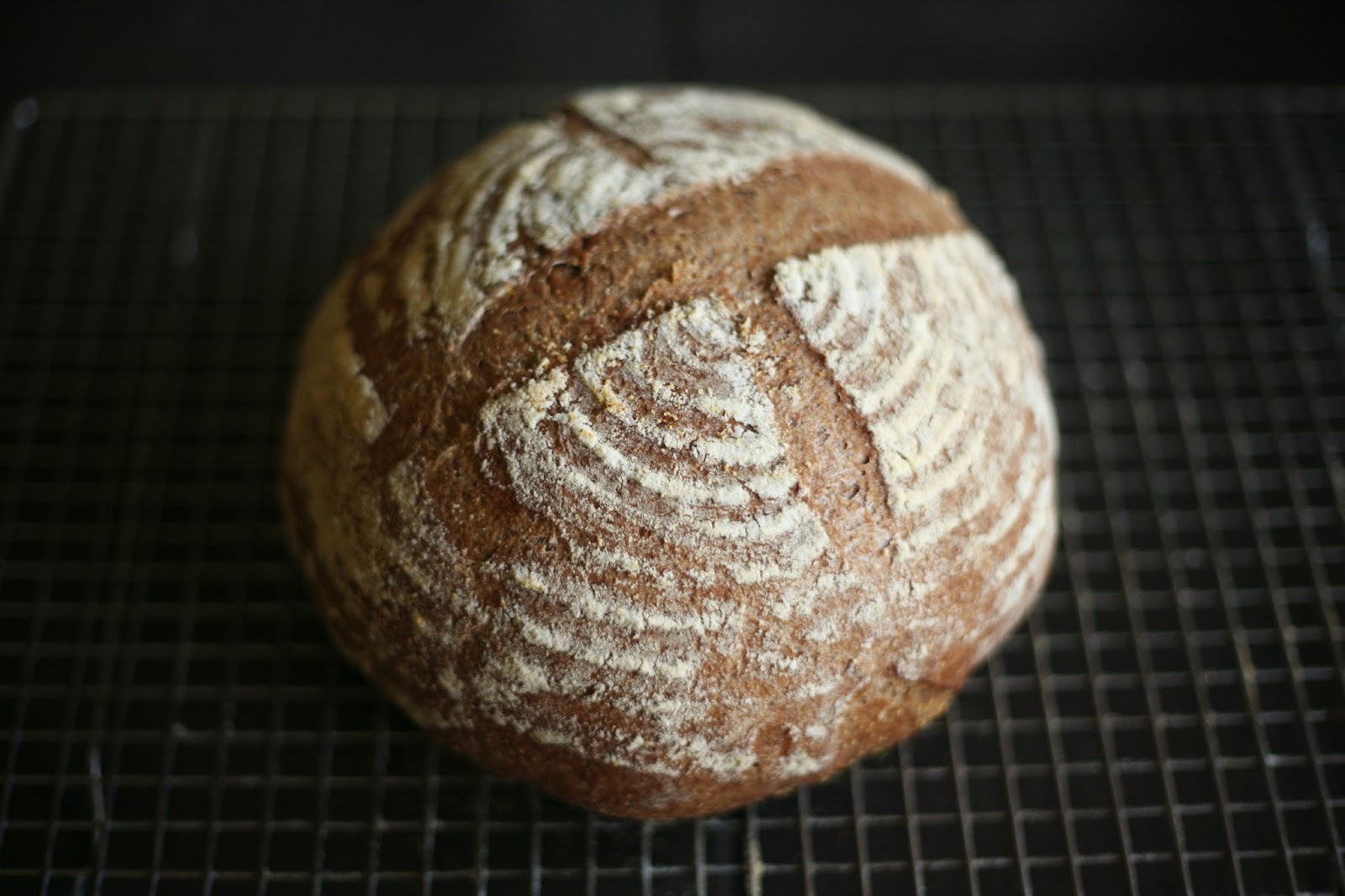The photograph showcases a beautifully baked round boule loaf of bread, resting on a cooling wire rack with a grid-like pattern that is mostly blurred. The bread, positioned prominently at the center of the image, features an intricate crosshatch cut on its dark, deep wheaty brown crust, suggesting it might be made from whole wheat or sourdough. The crust's detailed markings reveal the dough's rise and proofing process, with concentric flour rings adding to its rustic appeal. The background is a stark black, which highlights the bread's texture and color. The lighting, coming from the right, accentuates the bread's crackling crust and flour-dusted surface, giving it a hearty, artisanal appearance.